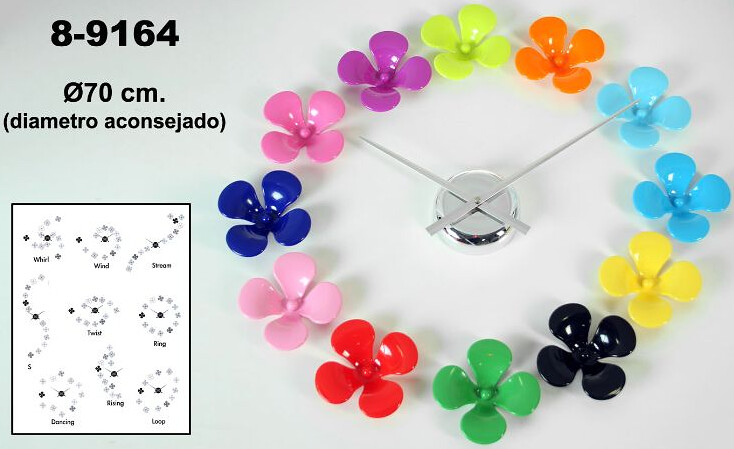This photograph showcases a distinctive and intricately detailed image. At the very top of the picture, there's a stark white background featuring black text that reads "8-916407CM." Just below, in black text against the white background, it states "DIA METRO ACO NSE JADO."

Further down, there is a black and white poster displaying an array of patterns and some accompanying text. Various words can be seen such as "whirlwind," "stream," "twist," "S ring," "rising," "dancing," and "loop," which likely describe different arrangements or designs. The beads depicted in these patterns seem to be organized meticulously.

The focal point of this photograph is the "ring" pattern prominently featured. This ring is composed of small, brightly colored plastic-looking flower decorations in a variety of hues including navy, light pink, purple, lime green, orange, light blue, darker blue, yellow, black, green, and red.

At the center of the ring pattern is a silvery clock face with two arms, creating a visual juxtaposition that adds an element of depth and complexity to the image. The overall composition is vibrant and textured, with each bead contributing to the detailed and visually captivating scene.